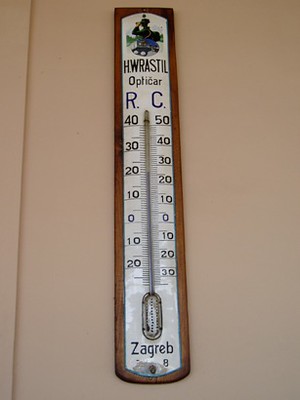A vertically oriented wall thermometer is mounted against a beige wall. The thermometer features a rectangular wooden frame. At the top of the thermometer is a small black statue, seemingly gazing into the distance. The inscription "H.W. Rastel Oblikar" appears in black letters at the center, while "Zagreb" is written at the bottom. The majority of the thermometer is occupied by a scale with dual measurements. On the left side, labeled "R," the scale ranges from 40 at the top to -20 at the bottom, in increments of 10. On the right side, labeled "C," the scale ranges from 50 at the top to -30 at the bottom, also in increments of 10. The scales are marked from top to bottom as follows: on the left under "R" – 40, 30, 20, 10, 0, -10, -20; and on the right under "C" – 50, 40, 30, 20, 10, 0, -10, -20, -30.